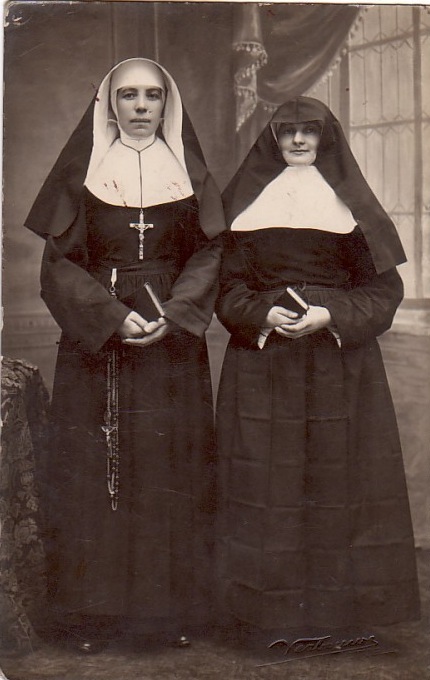In this aged black-and-white photograph, two nuns stand side by side, dominating the image from the bottom nearly to the top. Both are dressed in the traditional black habits and long gowns with white collars. Their heads are covered by black hoods, characteristic of their nun's attire. The nun on the left wears a prominent cross around her neck and possibly has a long strap hanging from her waist. Each nun holds a black book, presumed to be a Bible, with their hands folded in front of them at waist level. The nun on the right displays a faint smile, while the one on the left has a slight grin. Behind them, there's an open window with a curtain drawn to one side, revealing a thin glass pane. To the lower left side of the image, a table draped with a fancy tablecloth is partially visible, and the floor in the background appears dark. The overall grayish tone of the photo emphasizes its age.